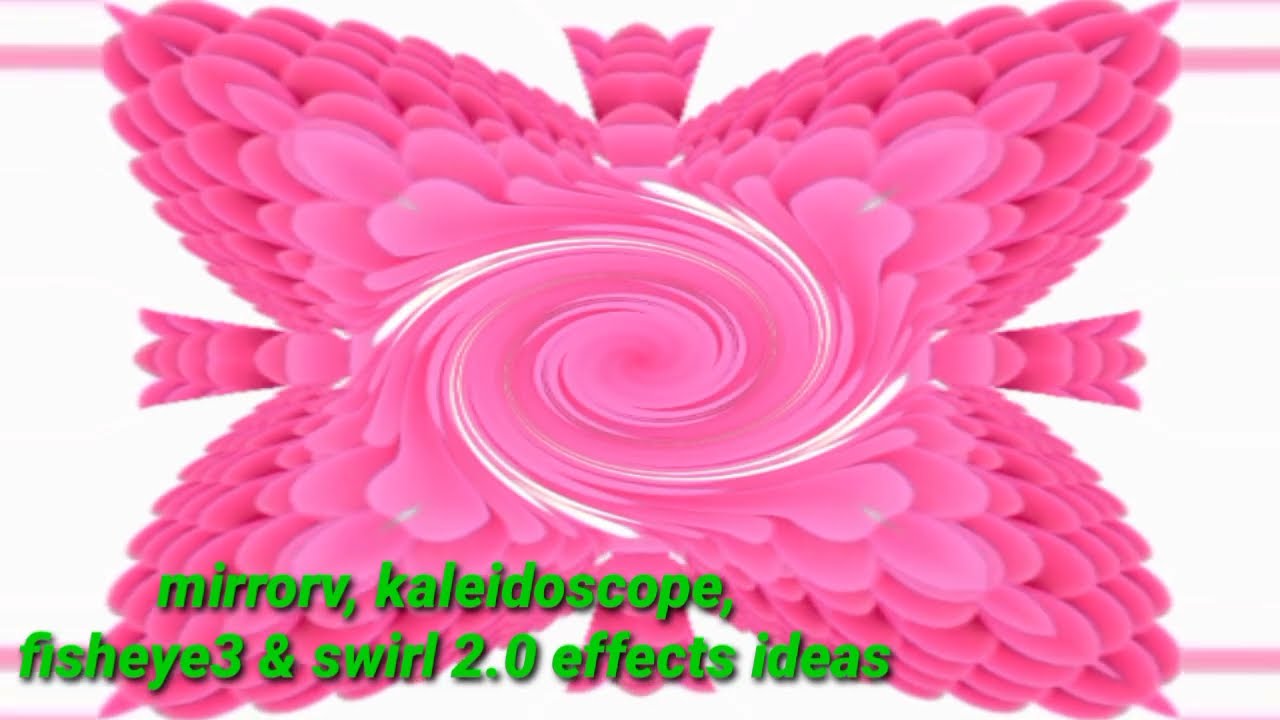The image features a vibrant, kaleidoscopic design against a white background, prominently showcasing a swirling, pink motif. At the center of the composition, a whirlpool of pink is interlaced with four white stripes, creating a dynamic swirl. This central swirl extends outward into multiple layers resembling elongated spade-shaped petals, which deepen in pink hue as they expand. The overall design forms a fluffy X shape, with pink crown-like structures at the top, bottom, and sides of the X. In the bottom left-hand corner, bright lime green text reads "Mirror V, Kaleidoscope, Fish Eye 3, and Swirl 2.0 Effects Ideas." The image evokes a sense of movement and fluidity, with elements that continuously collide and interact to create a mesmerizing visual effect.